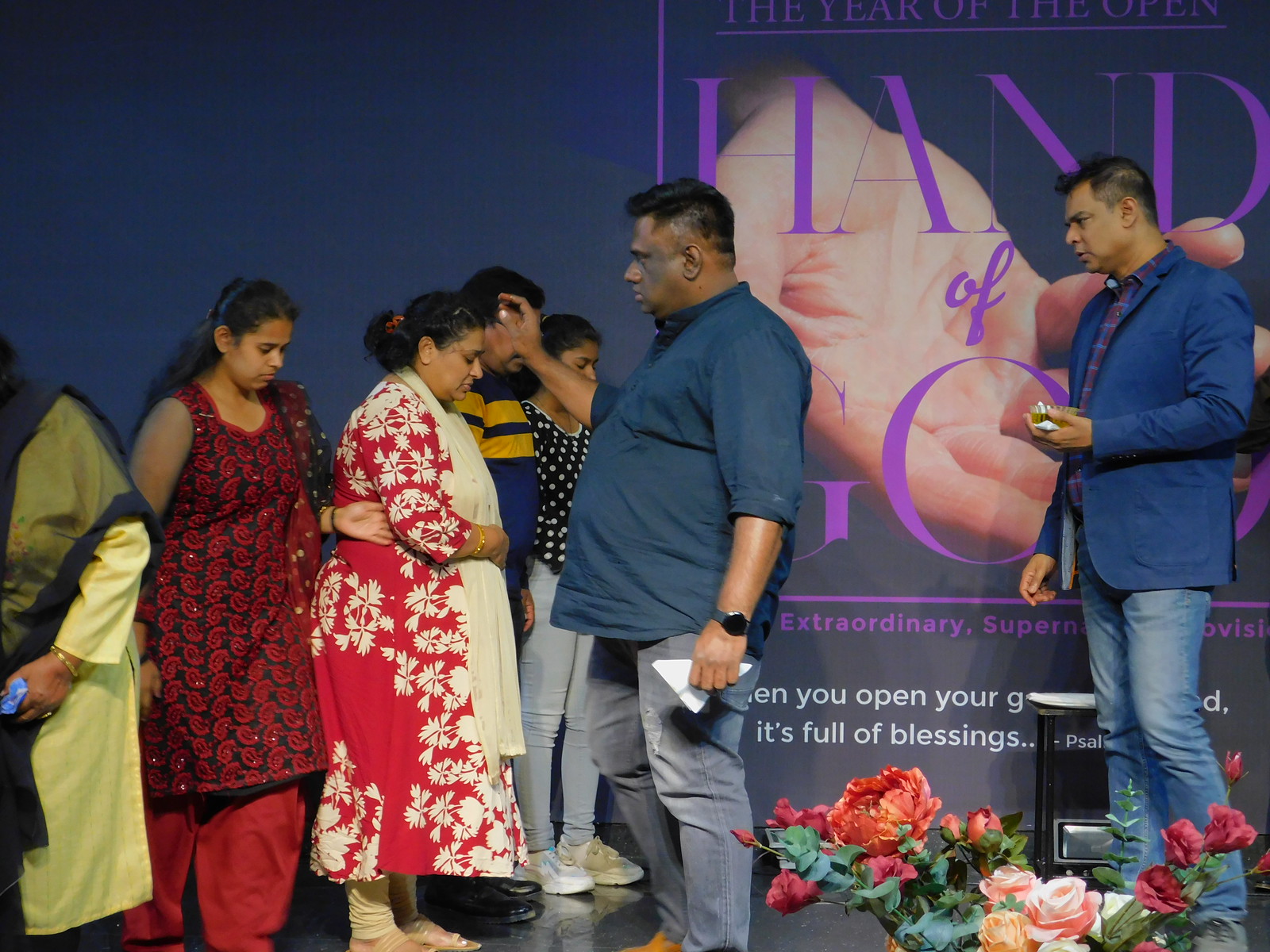In this color photograph, a religious event is taking place on a stage where a diverse group of people, primarily women of Asian Indian descent, and a few men are engaged in a prayer or blessing ceremony. Central to the image is a dark-skinned, heavyset man who appears to be a religious leader or pastor. He is wearing a dark blue button-down shirt, blue jeans, a black watch, and holds a white piece of cloth in one hand. With his other hand, he is hovering over the head of an older woman, blessing her as she stands with her eyes closed and head bowed. The woman is dressed in a red and white floral dress and a white scarf. Another woman behind her is in a red dress with a yellowish apron, and there's a younger girl in a black and red floral dress with red loose-fitting pants.

To the right in the image are two men: one is wearing a blue suit jacket over a checkered shirt with blue jeans and has a clean haircut, holding a cup or bowl; the other is assisting with the blessing. In front of them, pink, white, and green flowers add to the stage decor.

The backdrop features a large, blue poster with the faded text, "The Year of the Open Hand of God. Extraordinary," and a vivid image of an outstretched hand. The prominent signage, partially obscured by the participants, emphasizes the spiritual and healing theme of the event.